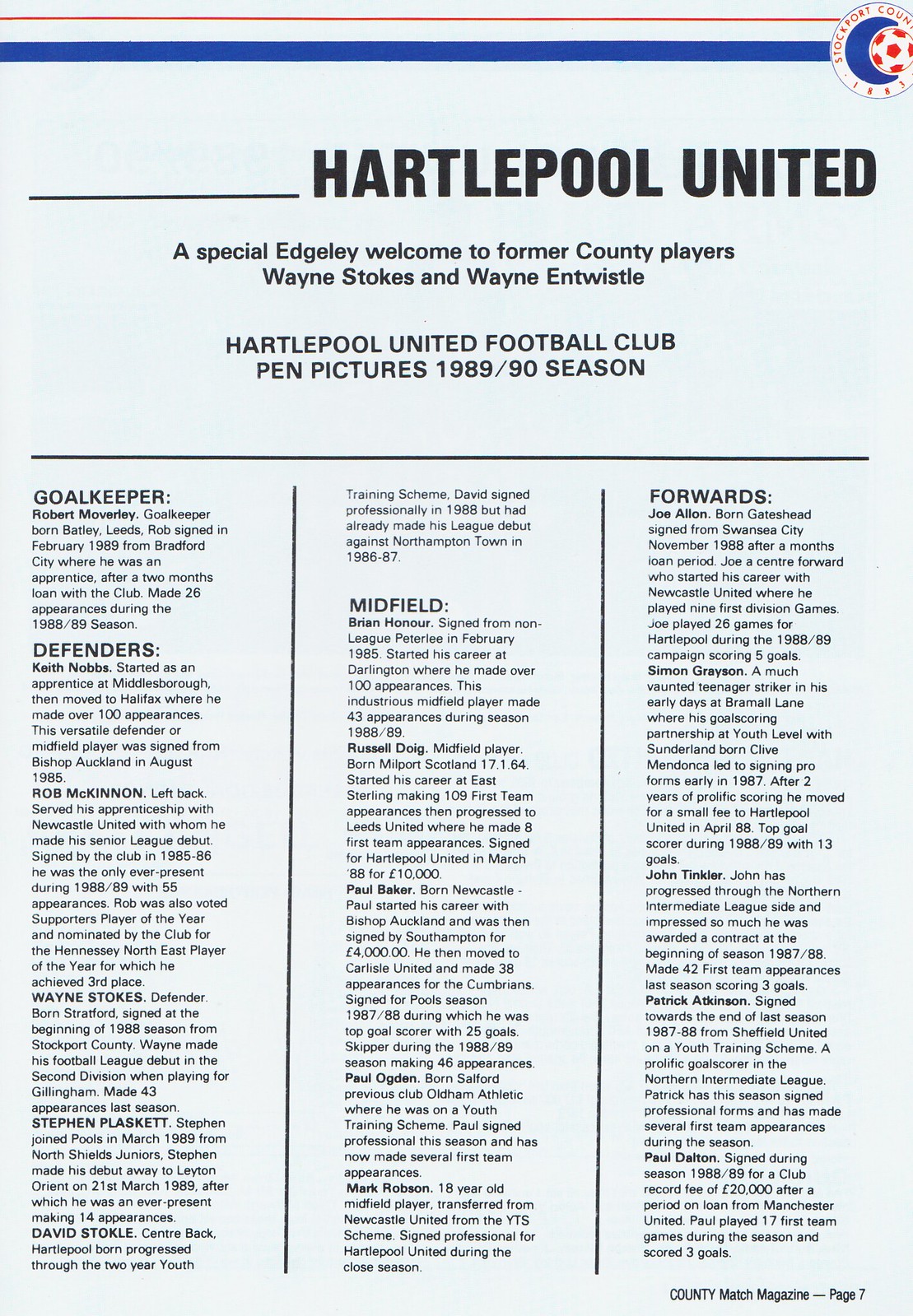The image is an official page from a soccer flyer, specifically designed on a light blue background with a layout that includes thin red and thicker blue horizontal lines at the top. On the upper right-hand corner, there is a circular emblem featuring a soccer ball over a blue interior, labeled with "Stockport County." The headline "Hartlepool United" appears prominently in large black capital letters beneath the lines, alongside smaller text welcoming former County players Wayne Stokes and Wayne Entwistle. Following this is the label "Hartlepool United Football Club, Penn Pictures, 1989-1990 season." 

A black line further down divides the page, which is filled with three vertical columns of detailed black text, each framed by vertical blue lines. The left column lists the "Goalkeeper," specifically Robert Mulverley, born in Batley Leeds, who signed from Bradford City in February 1989, accompanied by a brief biography. The "Defenders" section follows, enumerating players like Keith Knobbs, Rob McKinnon, Wayne Stokes, and Stephen Plaskett, each with extensive biographical details. The middle column is dedicated to the "Midfield" players, such as Brian Honor, Russell Dogue, Paul Baker, Paul Ogden, and Mark Robson, again with individualized biographies. The right column lists the "Forwards," including Joe Allen, John Tinkler, Simon Grayson, Patrick Atkinson, and Paul Dalton, each paired with thorough biographies. At the bottom right of the page, there is small, unreadable print and a note indicating this is "County Match Magazine, page 7."